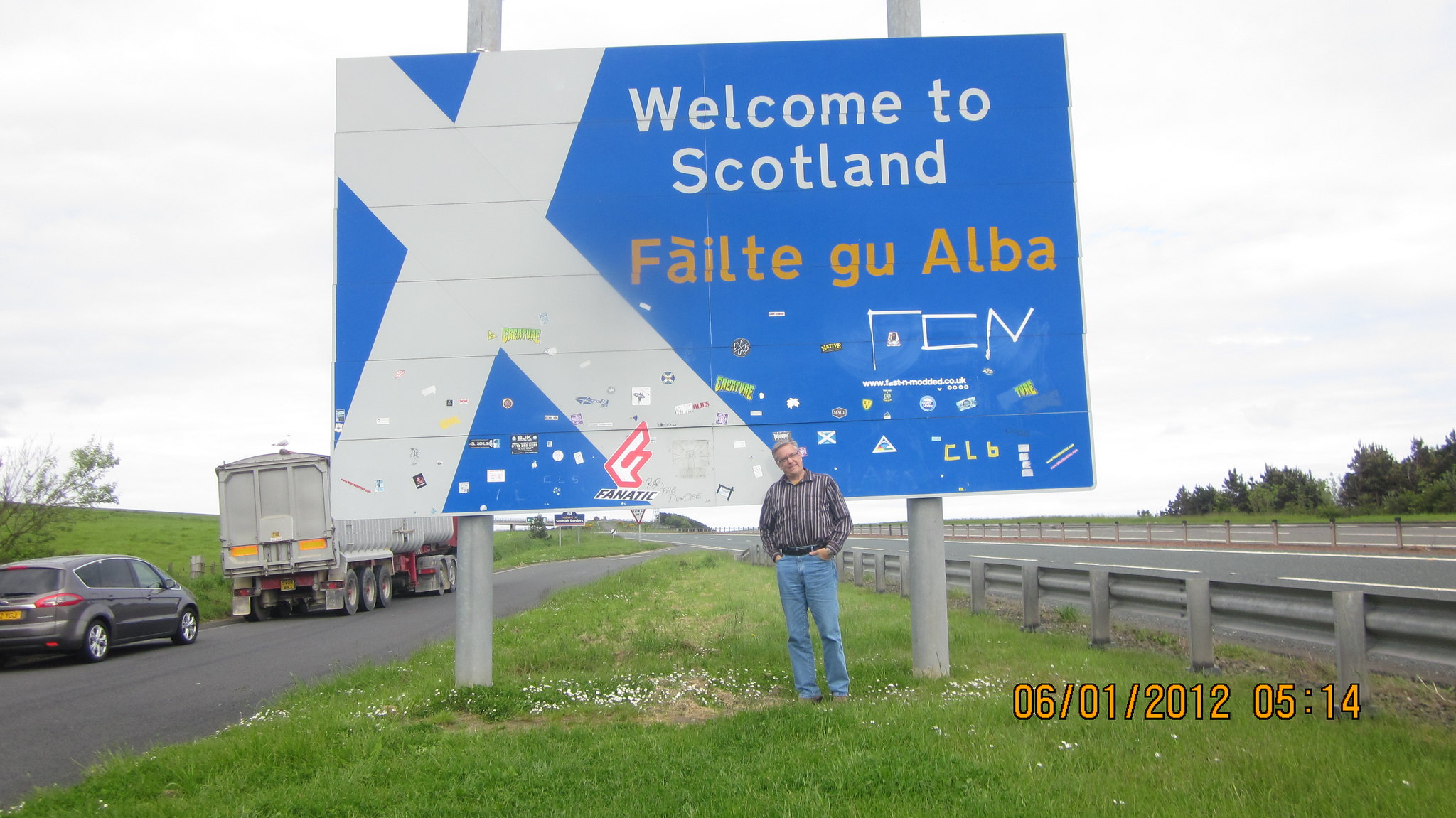In this image, a man in his 50s with gray hair, glasses, a blue and white striped long-sleeved shirt, and blue jeans stands posing in front of a large blue sign. The sign, situated between two roads—a small entry road on the left and a small highway on the right—features a prominent white X on the left side and reads "Welcome to Scotland" in white letters with "Fàilte gu Alba" in gold letters beneath. The sign is also adorned with numerous stickers from visitors over the years. Parked along the entry road are a gray car and a truck. Surrounding the scene is a grassy field to the left and a grove of trees in the distance on the right. A short gray fence lines the right-side road, which has a side barrier. The overcast sky casts a gray hue over the entire landscape. The date "06/01/2012" and the time "05:14" are noted at the lower right of the image.